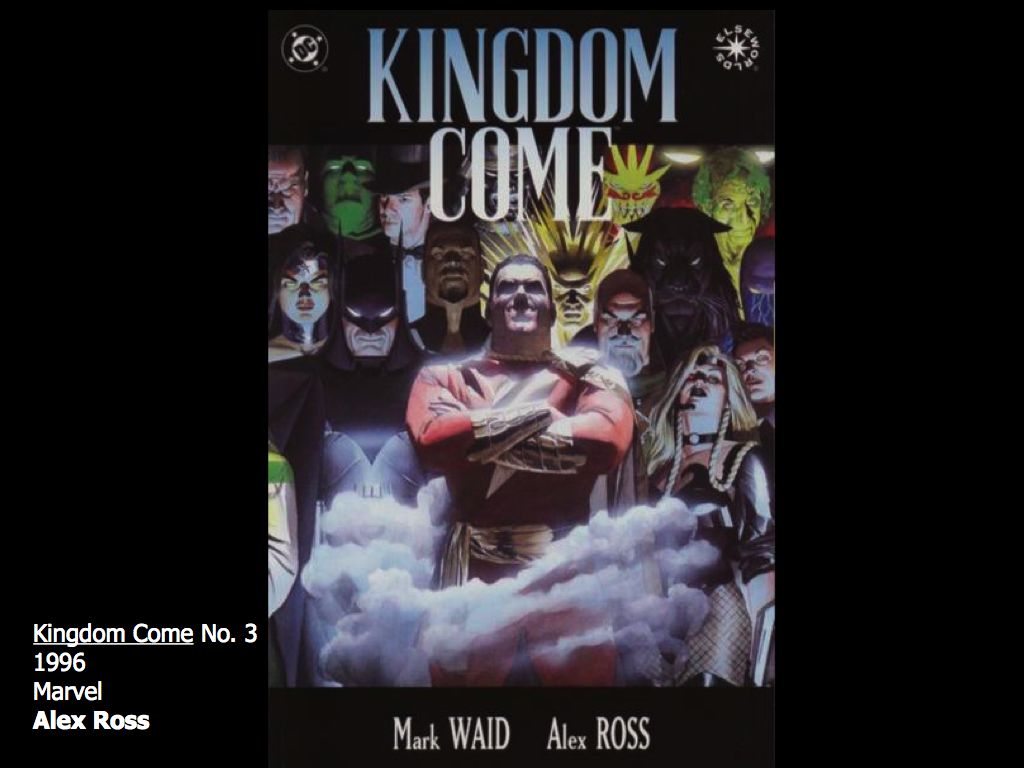A detailed caption for the image, merging elements from each description, would be:

"This is a digital artwork cover, possibly for a comic book or graphic novel, titled 'Kingdom Come,' prominently displayed at the top in large, all-caps white text with a blue gradient. The dark background enhances the dramatic effect of the cover. Flanking the title on either side are small circle logos: one says 'DC' and the other 'Elseworlds.' The artwork was created by Alex Ross in 1996 for DC Comics. The central image features an array of superheroes, including well-known characters such as Batman, Wonder Woman, what appears to be Iron Man, and a character resembling the Hulk. The image is densely packed with at least 13 characters, each rendered in a dark, gothic style. Notable details include Batman with smoke rising from his chest, a woman in a black jersey with a contorted face, and a character in a red suit with gold stripes that might be the Flash. At the bottom, it is captioned 'Kingdom Come Number 3, 1996, Mark Waid and Alex Ross,' underscoring the collaboration between the writer and artist."

This caption integrates the repeated elements and details shared across the descriptions, providing a comprehensive and detailed overview of the image.